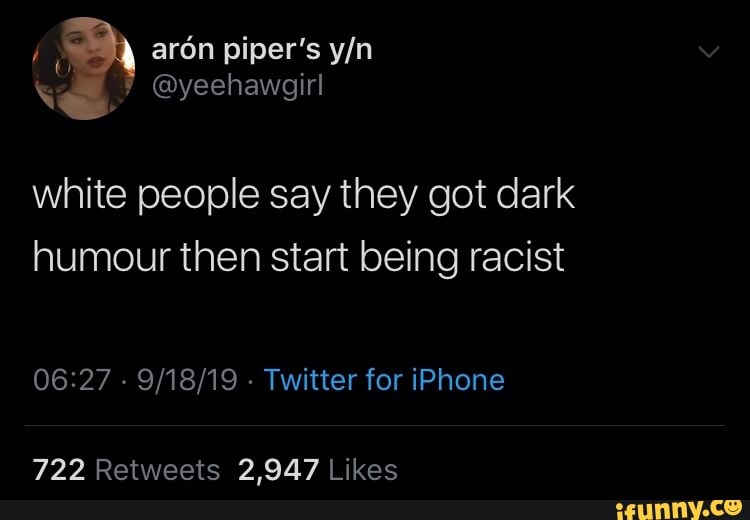This is a detailed description of a screenshot of a tweet.

The screenshot depicts a tweet featuring a predominantly black background. In the top left corner, there is a circular profile picture of a woman. The image shows her from just below her neck to the top of her head. She has long black hair cascading down both sides of her face, large gold hoop earrings, and her head is slightly tilted to the left. Her lips are visibly thick, and there is a subtle hint of sunlight to her right side. Adjacent to the profile picture, on the right, the name "Aaron Piper's Y/" is displayed, followed by a greater-than sign pointing downwards. Beneath this name, in smaller white text, is her handle, "@yee-haw girl."

The tweet text reads: "White people say they got dark humor then start being racist what?" Below the tweet, there is a timestamp in gray text that reads "6:27 PM · 9/18/19" with a small blue dot next to "Twitter for iPhone."

A horizontal gray line spans across the screenshot, under which the tweet's engagement metrics are displayed. Bold white text indicates "722" retweets and "2947" likes. At the bottom, a thin dark gray strip runs horizontally, with an off-yellow "iFunny.co" logo, where the 'o' in '.co' is stylized as a smiley face.